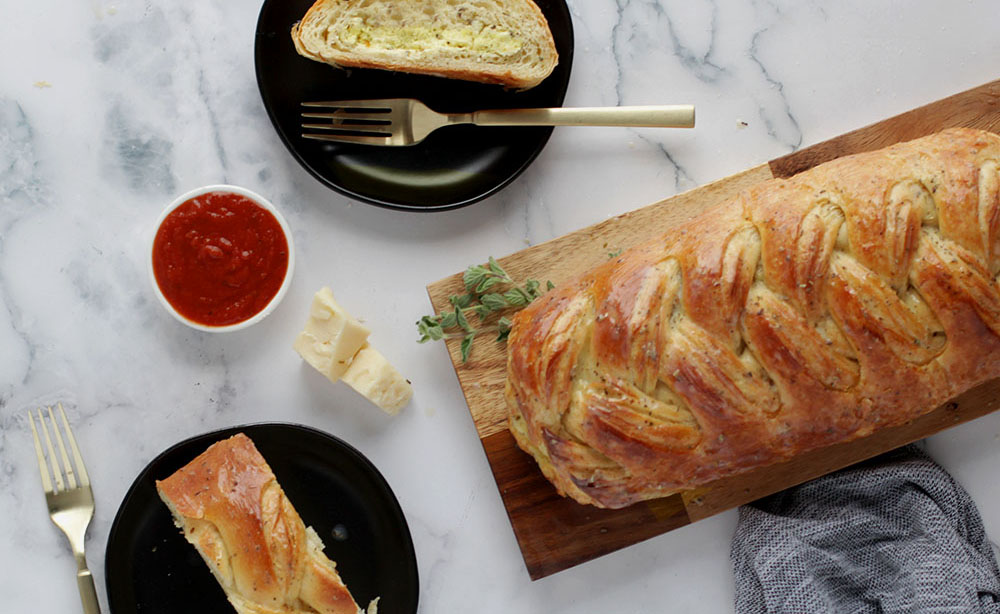The top-down photograph captures a meal laid out on a white marble table or countertop. Dominating the composition is a wooden breadboard with a whole, unsliced loaf of braided or garlic knot bread, garnished with a sprig of thyme or parsley. Towards the top left, a black plate features a buttered slice of bread with a fork resting horizontally across its edge. Nearby, a small dish of what appears to be marinara sauce or possibly ketchup adds a pop of color. Below this plate, another black plate holds another slice of bread. Situated between these two black plates, two small chunks of what might be cheese or butter sit invitingly. The setting evokes a rustic yet elegant meal presentation, enhanced by the interplay of textures and colors on the marble surface.